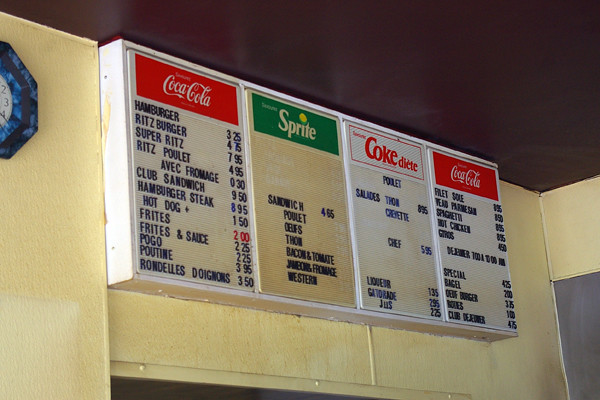The image captures a menu at what appears to be an old diner, evoking a nostalgic ambiance. The upper section of the image reveals a portion of the diner's interior, showcasing a smoothly finished brown ceiling. The wall is painted a warm beige color. On the left side of the image, there's a partial view of an analog clock with a dark blue octagonal frame adorned with a line through it, displaying the numbers 2, 3, and 4.

The menu itself comprises four panels, each highlighted with a colored bar at the top, indicating different soda brands. The first panel features a red bar with "Coca-Cola" written on it. The second panel has a green background with the Sprite logo, accompanied by a small lemon graphic. The third panel shows "Coke Diet" with a white label and a red border. The fourth panel, similar to the first, displays "Coca-Cola" with a red background and white text.

Below these headers, the menu lists various food items with prices:
- Hamburger: 3,25 €
- Ritz Burger: 4,25 €
- Super Ritz: 7,95 €
- Ritz Poulet: 4,95 €
- Avec Fromage: 0,30 €
- Club Sandwich: 9,50 €
- Hamburger Steak: 8,95 €
- Hot Dog: 1,50 €
- Frites: 2,00 €
- Frites and Sauce: 2,25 €
- Pogo: 2,25 €
- Poutine: 3,95 €
- Rondelles d'Oignon: 3,50 €

Given the presence of French text on the menu, it suggests that this diner might be located in a French-speaking region, likely in France.